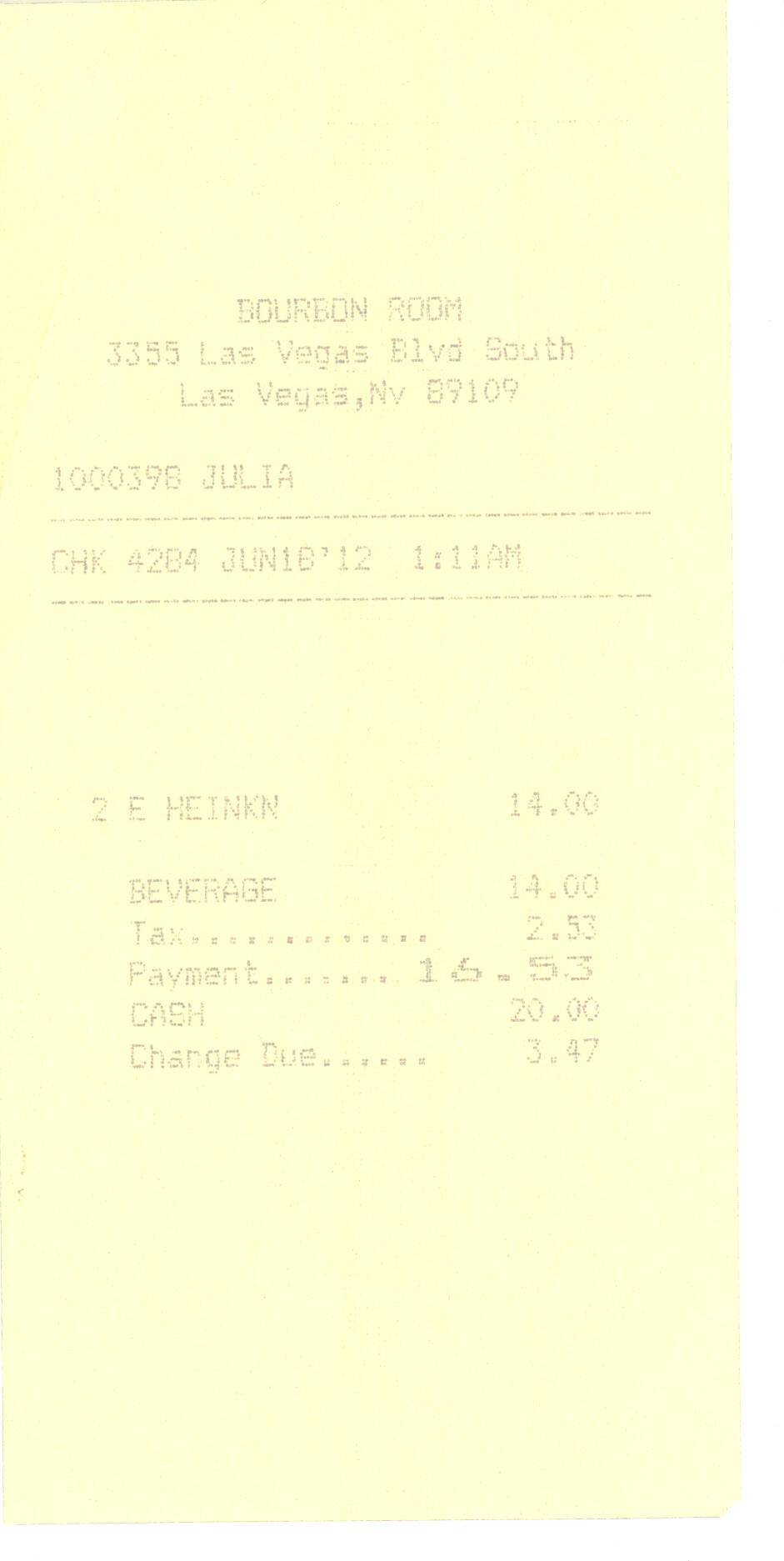The image shows an off-white, slightly yellowish receipt from the Bourbon Room, located at 3355 Las Vegas Boulevard South, Las Vegas, Nevada, 89109. The receipt number is 10000398, and it was issued by Julia. Detailed on the receipt is a Check (CHK) number 4284, dated June 18 at 1:11 AM. Items listed include a Heineken priced at $14.30 and a fairway priced at $14.30. The tax amount is $2.53, bringing the total payment to $16.53. The payment was made in cash with a $20 bill, resulting in a change of $3.47 returned to the customer.